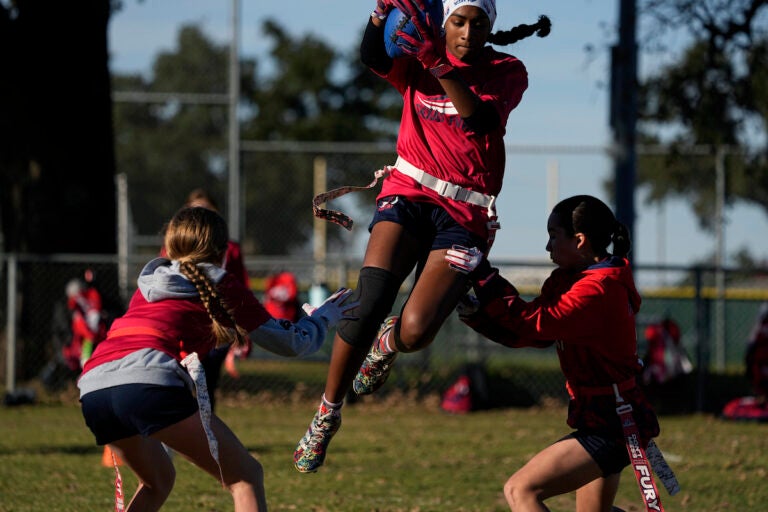In this vibrant real-life photograph, a heated flag football game is taking place on a grassy athletic field, set against a backdrop of a clear blue sky, green trees, and a tall silver wire mesh fence. The central figure, an African-American teenage girl with braided hair pulled back into a ponytail, is captured mid-air, having just leapt to catch a blue football. She is wearing a bright red jersey, blue shorts, and colorful rainbow sneakers. A knee brace adorns her right leg, and a belt with tassels labeled 'Fury' is cinched around her waist, her flags still intact.

To her left, a fair-skinned girl with long blonde pigtails, also outfitted in a red jersey and blue shorts, crouches with knees bent, reaching out to grab one of the center player’s flags. She has both her flags still attached.

On the right, another competitor, an Asian-American girl dressed in the same team attire, is reaching for the center player's other flag while placing a hand on the center player's thigh for balance. All three athletes are focused and intense, exemplifying the spirit and competition of the game.